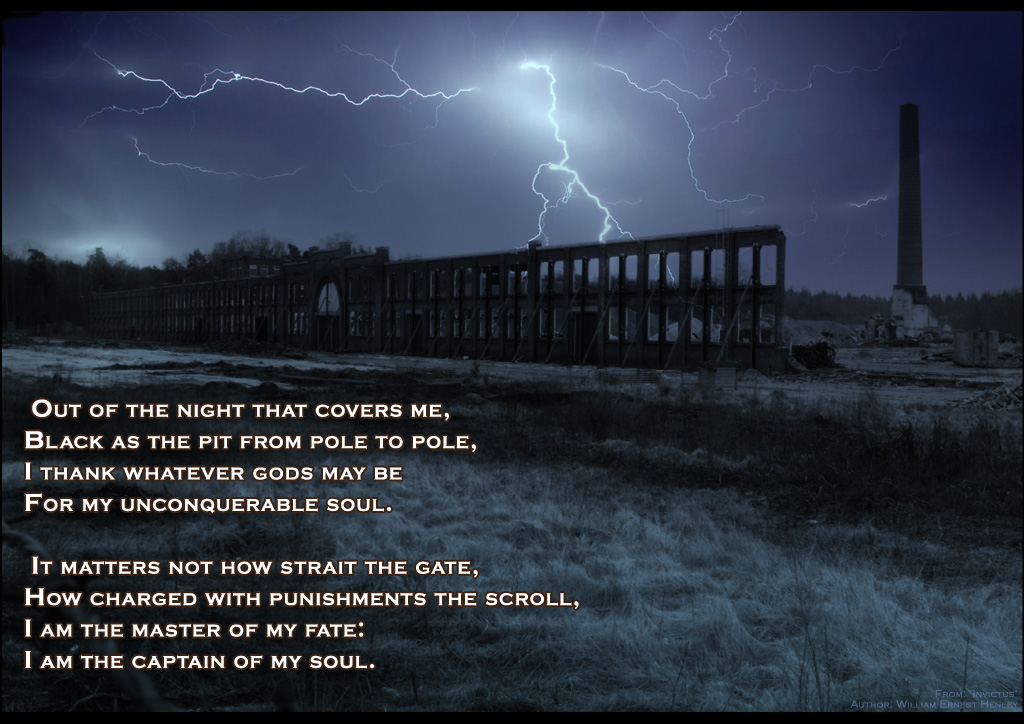The image portrays a dramatic and darkly atmospheric scene featuring a ruined factory with only its front facade still standing. The sky above is an ominous dark purple, dramatically lit by a large white lightning bolt striking the ground in the center. The ground appears to be covered in snow, extending across what seems to be a deserted, snow-covered yard. There is a hint of distant hills and a semblance of a destroyed tower to the left side. A stone fence is visible, adding to the desolate feel of the scene. In the bottom left corner, there are two paragraphs of white text, written in tidy lines. The text is a classic piece of poetry, reading: "Out of the night that covers me, black as the pit from pole to pole, I thank whatever gods may be for my unconquerable soul. It matters not how straight the gate, how charged with punishments the scroll. I am the master of my fate. I am the captain of my soul." The entire scene is both haunting and inspirational, combining the grim setting with powerful words of resilience.